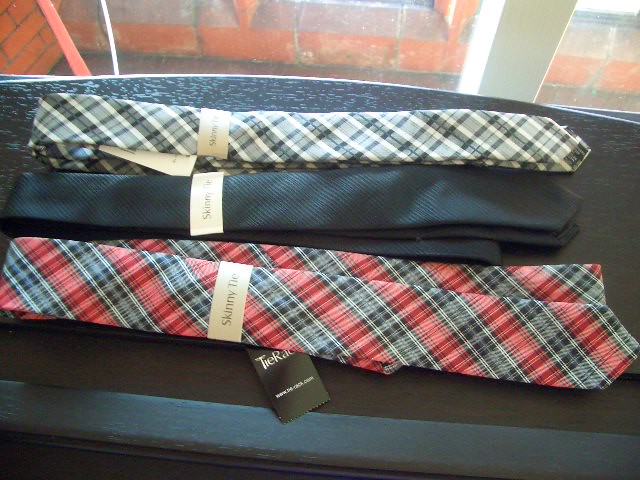A photograph captures three brand new men's skinny ties neatly arranged on a dark wooden table, positioned near a window that allows daylight to illuminate the scene, offering a glimpse of red brick walls outside, suggesting a residential setting. The ties, identified by their tags as being from Tierack.com, are uniformly packaged with white labels that read “skinny tie.” The bottom tie features a red, black, and white plaid pattern. The middle tie is solid black with textured stripes offering a subtle sheen. The top tie sports a white, black, and gray plaid design. The meticulous arrangement and pristine condition of the ties, combined with the tags and packaging, suggest they might have just been purchased or are part of a product display.